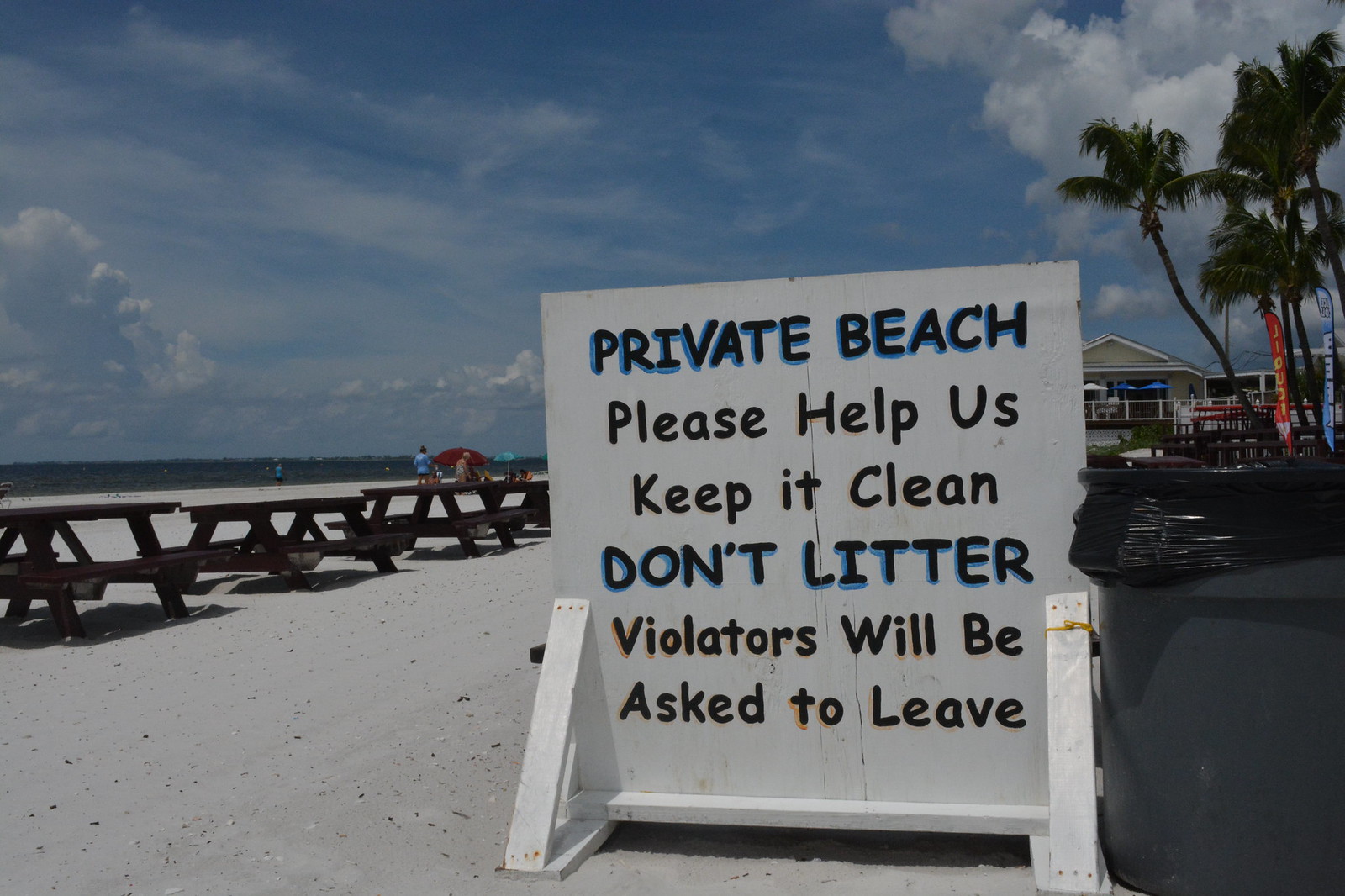This photograph captures a vibrant beach scene characterized by its white sandy surface. Prominently positioned in the center is a large white sign held up by wooden planks, which reads: "Private Beach" in bold blue letters at the top, followed by "please help us keep it clean" in red letters, "don't litter" in larger blue letters, and "violators will be asked to leave" in smaller red letters. To the right of the sign, a gray trash can with a black lid stands ready to keep the beach tidy. To the left, several wooden picnic tables stretch from the center toward the background, where a handful of beachgoers and umbrellas can be spotted. Further beyond, the sea meets a striking blue sky adorned with fluffy white clouds. In the background to the right of the sign, a structure surrounded by palm trees, likely a house or a business, completes the serene yet lively scene of this private beachfront area.